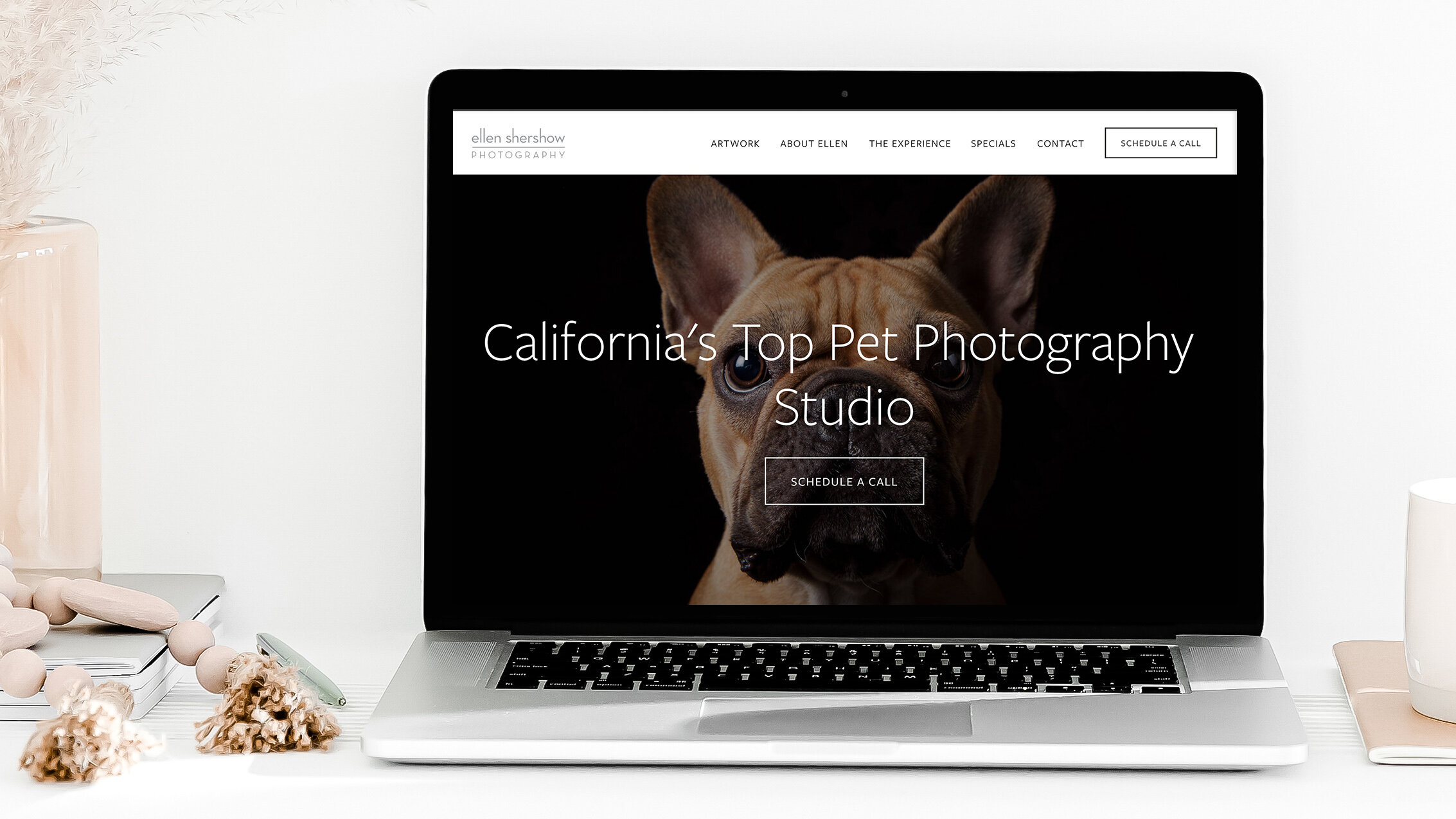The photograph presents a clean and minimalist workspace with a focus on elegant simplicity. Set against a pristine white background, likely a wall, a white table stretches across the lower portion of the image. 

On the table's surface, a range of carefully selected items is neatly arranged. To the left, there's a stack of white and gray books that provide a monochromatic touch. A tall, beige vase filled with complementary beige plants adds a natural and warm accent. Resting next to the vase are decorative beads with tassels, contributing a soft, tactile element to the scene. Additionally, a sleek silver pen lies poised and ready for use.

The centerpiece of the tableau is an open silver laptop with black keys. The screen prominently displays the website "Ellen Shensho Photography." The page features various navigational elements such as "Artwork," "About Ellen," "The Experience," "Specials," "Contact," and a prominent "Schedule a Call" button. A vibrant photograph of a tan French bulldog with a black muzzle is displayed prominently, alongside the text "California's Top Pet Photography Studio."

To the right side of the table, a small pink book adds a subtle pop of color, complemented by a white mug sitting atop it, presumably ready to offer refreshment to the person behind this serene and efficient workspace.